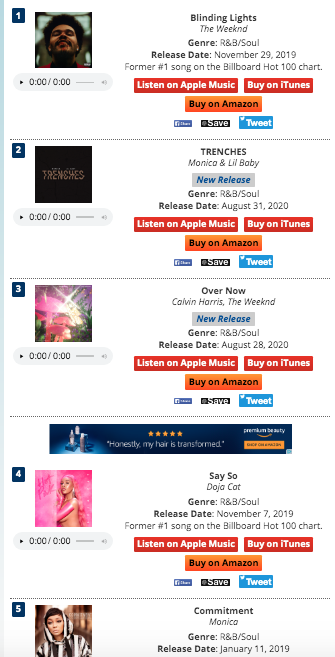This website features a comprehensive selection of music available for listening or purchase on iTunes, Apple Music, and Amazon. The user interface categorizes tracks by popularity and genre, providing multiple interaction options including purchasing, tweeting, or saving songs.

1. **Blinding Lights by The Weeknd**
   - **Genre:** R&B
   - **Release Date:** November 29, 2019
   - **Formerly Ranked:** Number one on the Billboard Hot 100 chart
   - **Description:** The Weeknd, an African American artist known for his distinctive dreadlocked hair, is pictured looking upwards. Available purchase options are highlighted – red for iTunes, orange for Amazon – alongside share buttons including a blue Twitter icon.
   
2. **Trenches by Monica and Lil Baby**
   - **Genre:** R&B
   - **Status:** New Release
   - **Description:** A collaboration featuring Monica and Lil Baby. The promotional icon showcases a black box with the word "Trenches." Availability options mirror the previous entry, with Apple Music, iTunes, and Amazon as purchasing platforms, and a Twitter icon for sharing.
   
3. **Over Now by Calvin Harris and The Weeknd**
   - **Genre:** R&B
   - **Release Date:** August 28, 2020
   - **Status:** New Release
   - **Description:** The icon depicts mushrooms against a space galaxy backdrop. This song combines Calvin Harris’s production with The Weeknd’s vocals. Purchase options and social media buttons are consistent, featuring red and orange boxes for iTunes and Amazon purchases, respectively.
   
4. **Say So by Doja Cat**
   - **Genre:** R&B
   - **Release Date:** November 7, 2019
   - **Formerly Ranked:** Number one on the Billboard Hot 100 chart
   - **Description:** Doja Cat, shown sideways against a pink background, appears to be nude with pink paint on her arm. Interactive options include purchasing through Amazon, tweeting, or saving, and possibly Facebook sharing.
   
5. **Commitment by Monica**
   - **Genre:** R&B
   - **Release Date:** January 11, 2019
   - **Description:** Monica is pictured wearing a striped hooded shirt. The song currently holds the fifth position, with standard purchase and share options provided.

Overall, the website effectively curates popular and new R&B releases with clear, visually distinct icons for purchasing and sharing on social media platforms.